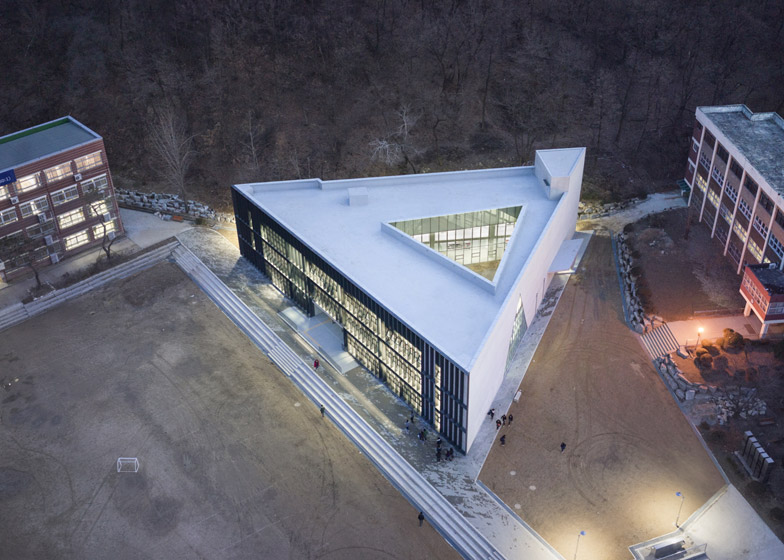This is a horizontal, rectangular night-time aerial photograph taken from a tall building or drone. At the center of the image is a distinctive, white triangular building featuring an inner courtyard filled with light. The front facade, primarily made up of windows, is illuminated with unreadable writing on the left. There is a door for entry, while the left side of the triangle has numerous windows, and the right side remains blank and purely white. Notably, the roof has a triangular window offering a view from above. Surrounding the central building, on the left stands a well-lit square-shaped, brick building with a lot of windows, and to the right, another building with minimal or no lights visible. The area between these buildings is dominated by concrete, sporadically interspersed with outside lights and a visible staircase leading to the building on the right. The background showcases dark, numerous trees and a road lying in front of the triangular building, framing this unique urban landscape filled with many buildings, roads, and lights.